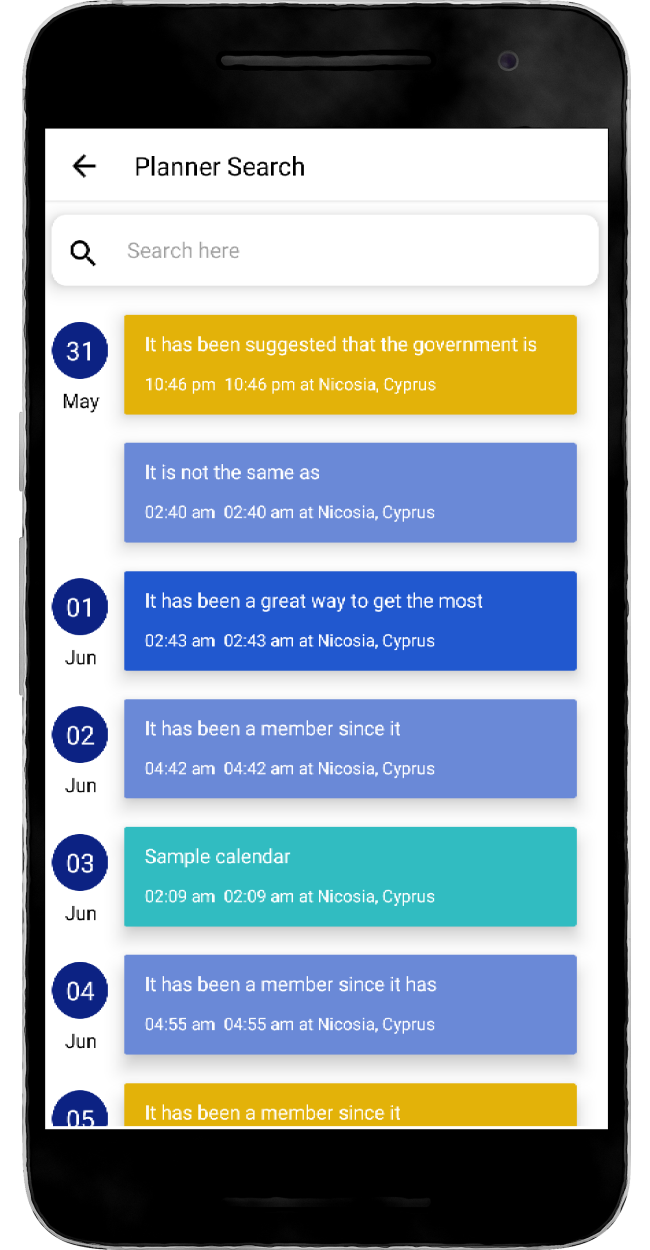The image depicts a mock-up of a cell phone screen. The phone features a black bezel along the top, bottom, and sides of the display. At the top of the screen, within a white area, there is a black arrow. Alongside it, in white text, the words "Planner Search" are displayed. Beneath this text, in a white rectangle with rounded corners, there is a black magnifying glass icon with the phrase "Search here" in gray inside it.

On the left, surrounded by an arrangement of differently colored rectangles, there is a blue circle with white numbers reading "31". Below this, it is written in black, "May". Next to it, an orange rectangle with white text states, "It has been suggested that the government is," followed by the timestamp "10:46 PM" and location "Nicosia, Cyprus".

Another mid-blue rectangle beneath it displays "It is not the same as," followed by "02:40 AM". This is also marked at "Nicosia, Cyprus". Next, there's a dark blue circle indicating "01" with "JUN" (June) written below it. The message following this indicates, "It has been a great way to get the most," sent at "2:43 AM" from the same location.

The screen continues to the 2nd of June, highlighted by a mid-blue rectangle with white text stating, "It has been a member since," timestamped "4:42 AM". Following this is another dark blue circle marked "03" with "June" beneath it. Adjacent to it, a teal rectangle in white text reads, "Sample calendar" with a time of "2:09 AM".

Finally, a dark blue circle marked "04" with "June" below it is shown, alongside a mid-blue rectangle in bold white text saying, "It has been a member since," and timestamped "4:55 AM". The last element visible is a dark blue circle with "05" in white; outside this circle, within an orange rectangle, bold white text reads, "It has been a member since," though this phrase is cut off in the image.